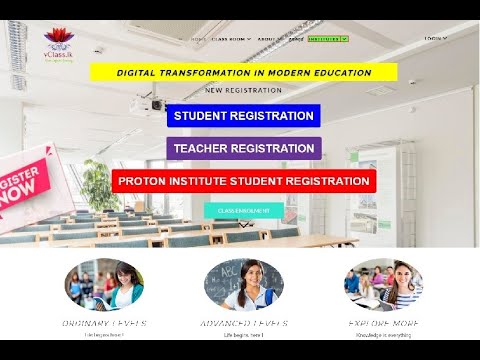The image outlines modern educational themes centered on digital transformation, all framed with a classroom background featuring numerous tables and chairs. At the top, bold black text reads "Digital Transformation and Modern Education" inside a prominent yellow rectangle. Below, three distinct registration options are prominently highlighted: "New Registration" in white text on a purple rectangle, "Student Registration" in white text on a blue rectangle, and "Teacher Registration" in white text on a red rectangle. The mention of "Proton Institute Student Registration" also appears in white text, though the position isn't specified.

In the lower section, three circles are laid out, each depicting different educational scenes. The first circle is labeled "Ordinary" and showcases a girl engrossed in reading a book outdoors with a few people visible in the background. The second circle, labeled "Advanced," features a girl equipped with a book bag, standing in front of a chalkboard covered in mathematical writings. The third circle, labeled "Explore More," suggests further opportunities for educational engagement, though specific visuals related to this aren't described.